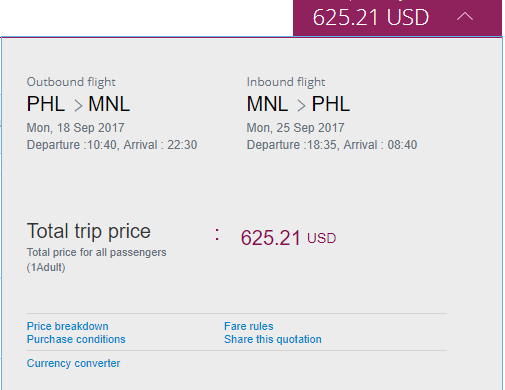This image depicts a web page displaying airline information. In the upper right-hand corner, there is a small, reddish-brown rectangle containing the text "625.21 USD" in white. Just below this, a large gray box outlines the flight details.

The first section within the gray box is labeled "Outbound Flight." It displays the route from "PHL" to "MNL" in uppercase letters, connected by an arrow. The flight date is specified as "MON, 18 SEP 2017." Departure and arrival times are listed as "Departure: 10:40" and "Arrival: 22:30."

To the right of this, another section titled "Inbound Flight" details the return route from "MNL" to "PHL," also indicated with an arrow. The return flight date is "MON, 25 SEP." The same date formatting and prominent labeling are used throughout for clarity.